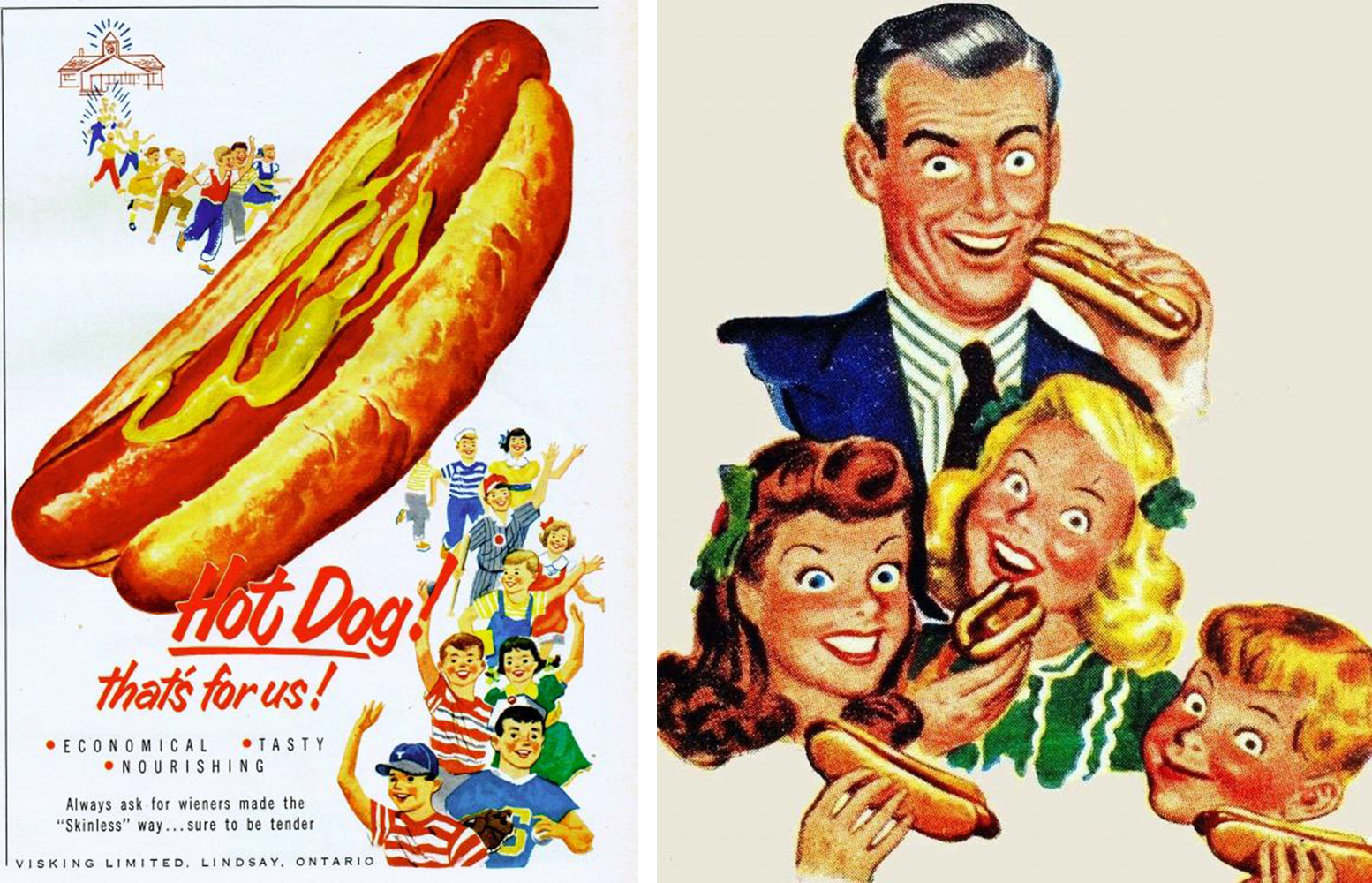This vintage advertisement from the 1940s or 1950s promotes hot dogs with cheerful illustrations and enticing text. On the left side, a single hot dog with mustard in a bun is prominently featured, angled from the bottom left to the top right of the image. Beside it, in bold red script, the slogan "Hot Dog, That's For Us!" stands out. Behind the hot dog, a parade of cartoon characters, including boys and girls in baseball uniforms and caps reminiscent of the 1940s, march exuberantly, suggesting a festive school event.

On the right side of the ad, a wholesome family scene is depicted: a father in a suit, a mother, and their two children—a boy and a girl—all smiling and eagerly holding hot dogs, looking delighted. This part emphasizes the family-friendly nature of the product. The ad touts the hot dogs as "Economical, Tasty, Nourishing," with red bullet points accentuating each quality. The text urges consumers to "Always ask for wieners made the skinless way, sure to be tender," and mentions the producer, "Visking Limited, Lindsay, Ontario."

Overall, the ad combines vibrant colors and joyful imagery to create a compelling and nostalgic appeal for "wieners made the skinless way," sure to be tender and enjoyed by families everywhere.